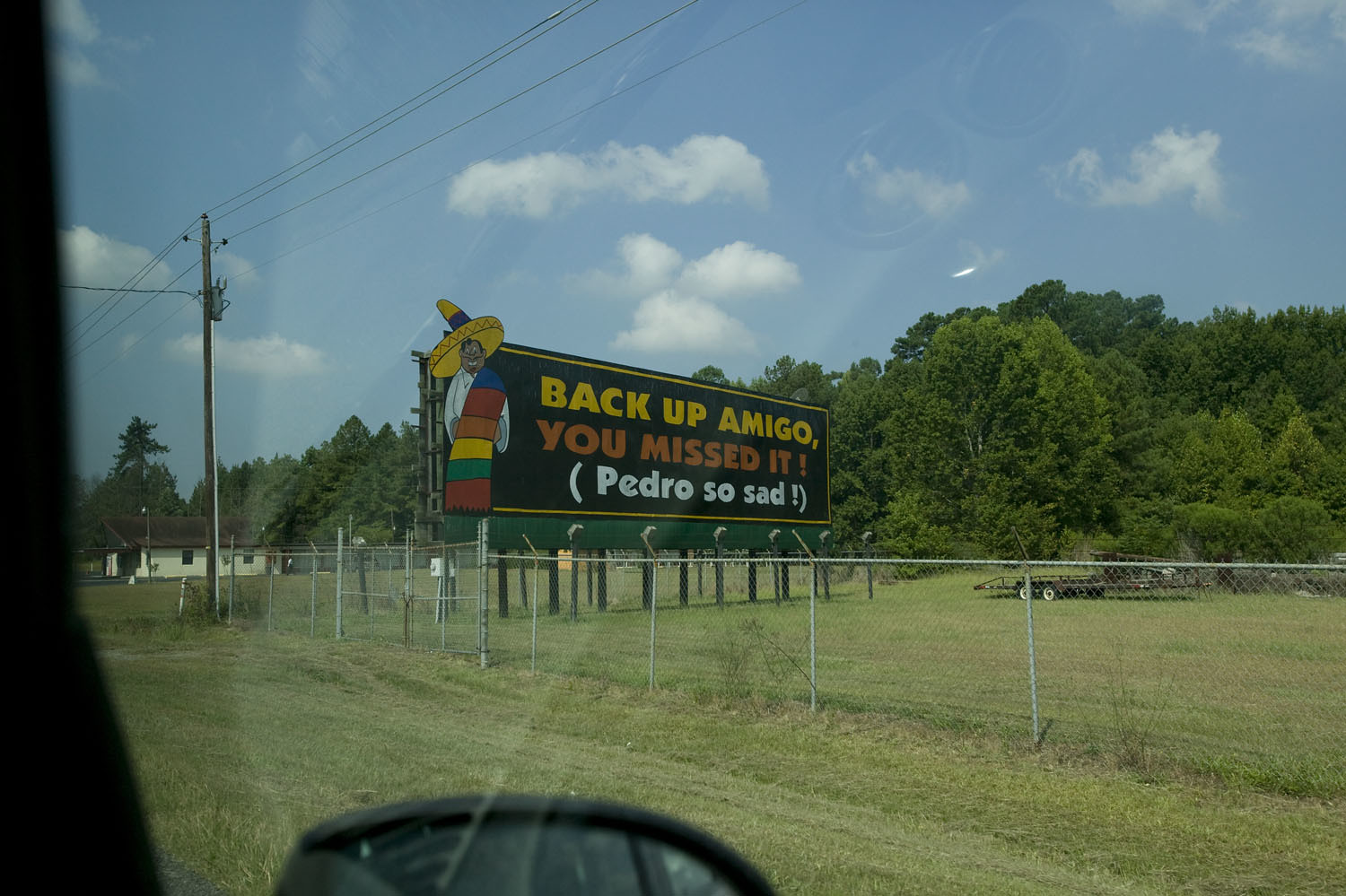This image captures a vividly detailed roadside sign. The sign itself is rectangular in shape and prominently displays a vibrant array of colors and texts. The primary message on the sign is divided into three distinct parts: 

- **"Backup Amigo"** is written in bold yellow lettering.
- **"You missed it!"** is highlighted in bright orange font.
- The phrase **"(Pedro so sad!)"** appears in white font within parentheses, emphasizing a sense of disappointment.

Additionally, the sign features an illustration of a tan-skinned man with traditional Mexican features. He is depicted wearing a yellow sombrero adorned with a purple and blue stripe. The entire sign is brightly illuminated by several lights aimed at it, ensuring its visibility. The sign is mounted on multiple short poles for support.

Enclosing the sign is a chain-link fence that separates it from the surrounding environment. The area around the sign boasts a meticulously maintained green lawn, contributing to the overall cleanliness and orderliness of the scene. The picture appears to have been taken from a vehicle, as suggested by the perspective and framing.